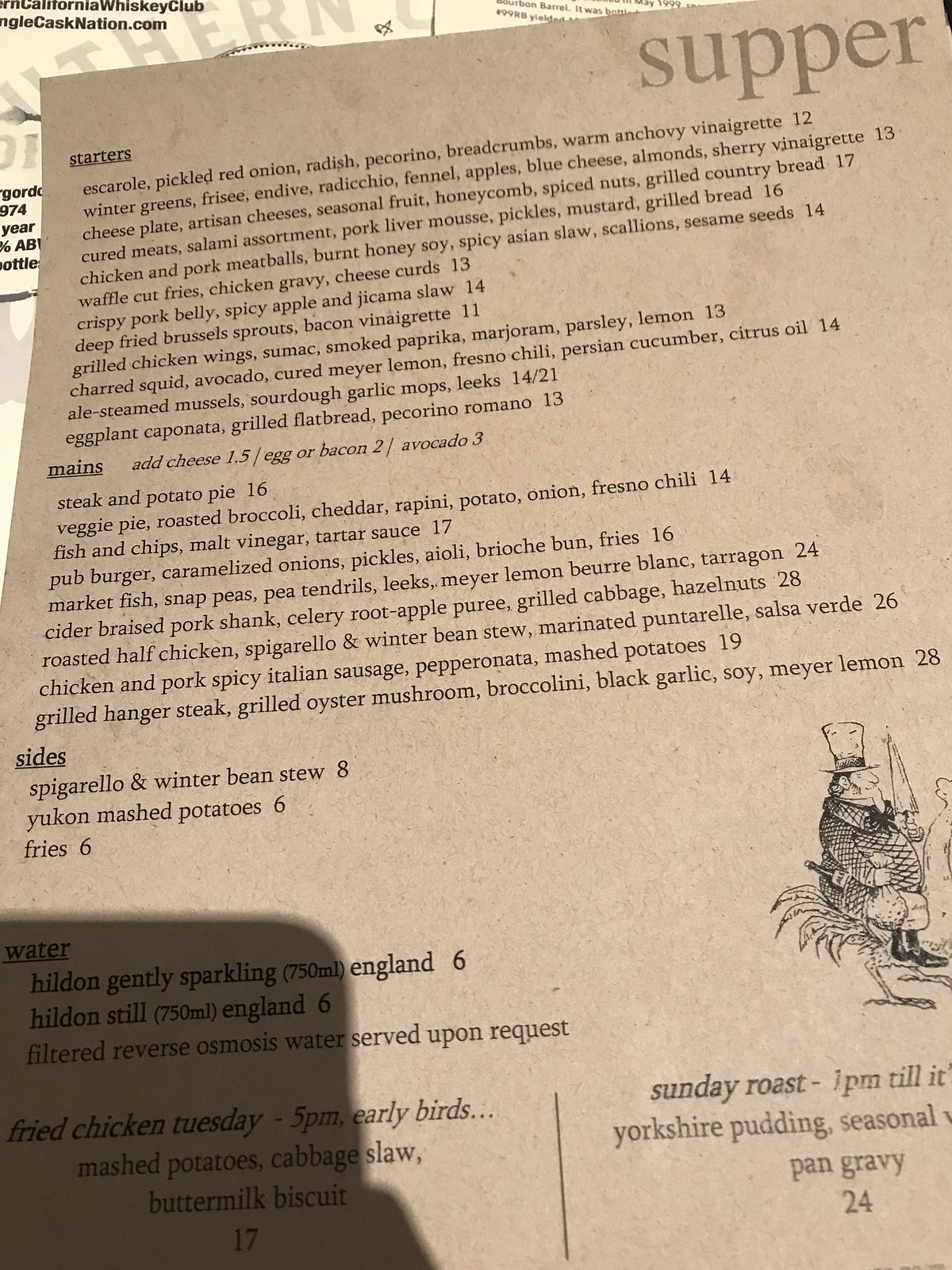The image displays a page from a restaurant menu printed on light brown paper. In the upper right corner, the word "Supper" is prominently featured in large gray font. The menu is neatly organized into sections, beginning with "Starters," which is underlined for emphasis. 

Under the "Starters" heading, the menu lists a variety of appetizers including:
- Escarole with pickled red onion, radish, pecorino, breadcrumbs, and warm anchovy vinaigrette, priced at $12.
- Winter greens such as fresh sea endive, radicchio, fennel, and apples.

The detailed list of starters continues extensively.

The "Mains" section, also underlined, follows and presents the main dishes. Notable entries include:
- Steak and potato pie.
- Veggie pie.
- Roasted broccoli combined with cheddar, rapini, potato, onion, and Fresno chili.

Towards the bottom of the menu, there is a section for "Sides," and notes mention "Water" and a special "Fried Chicken Tuesday."

The menu layout is clear and organized, providing a comprehensive list of the restaurant's offerings.